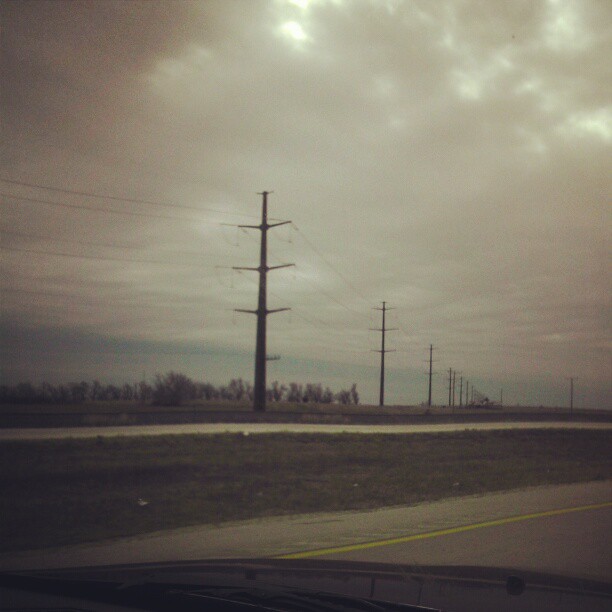In this photograph, we see a gloomy, overcast day along a two-lane country highway. The image, possibly taken from the driver's side of a car, reveals a monotonous row of tall utility poles stretching into the distance, each connected by power lines. The blurred and dark photo captures the edge of the car's front bumper in the lower right corner. On the left side of the photograph, a line of trees and short shrubs sits adjacent to the road, accompanied by patches of grass. Above, abundant cumulonimbus clouds dominate the sky, indicating potential rain. A slight blue haze in the distance might point to distant mountains. A single strip of yellow divider line is visible on the gray road. Despite some light shining through the clouds, the overall scene appears quite somber and dreary.